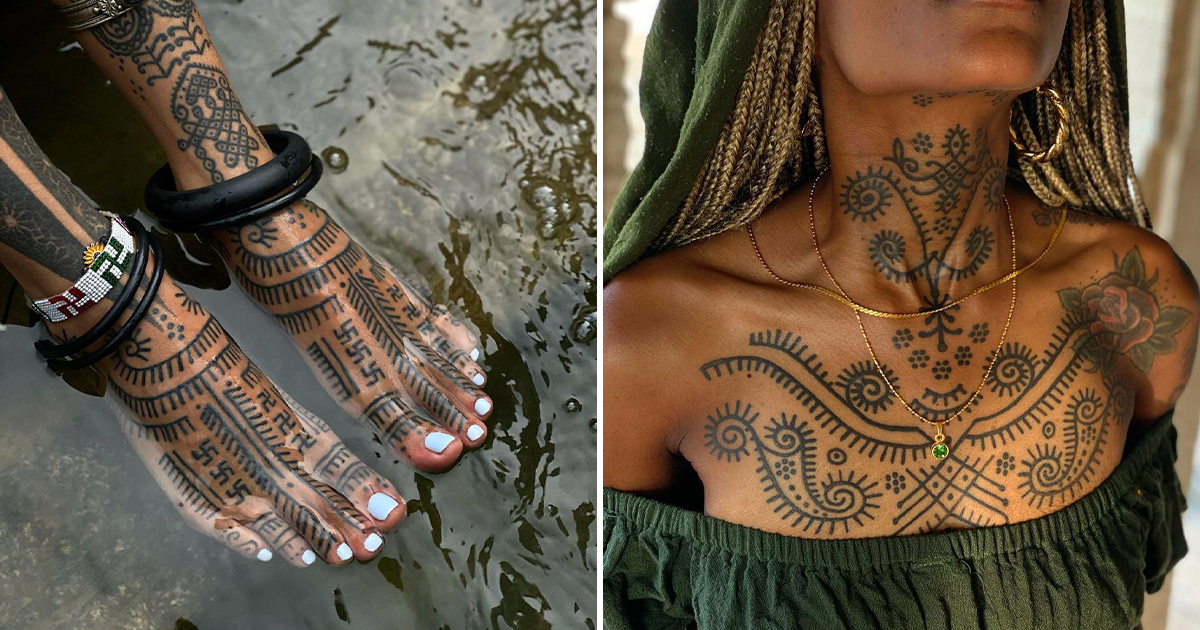The image is a split-screen composition featuring a black woman adorned with intricate tattoos. On the left, her feet are submerged in greenish water with visible stone beneath. The feet, shins, and calves display black, tribal line-work tattoos, with decorated white toenails and anklets: black cuffs and a white, green, and red band. Notably, swastika symbols are incorporated into the tattoos on her feet, referencing their historical significance prior to their appropriation by the Nazis. Her feet are angled diagonally from the top left corner. 

The right side of the image presents an upper body view of the same woman, or potentially a different woman with similar tattoos, from the upper lip to mid-chest. Her long, blonde braids frame her face, and she wears a green headscarf draping down her shoulders, complemented by large gold hoop earrings. She wears a dark green blouse or dress that is pulled down just above her bust, revealing a continuation of the black tribal tattoos across her chest and neck. Her head is tilted up, accentuating the tattoos' prominence. The photo, embodying photographic representational realism, highlights the detailed and culturally rich body art spanning across both segments of the image.